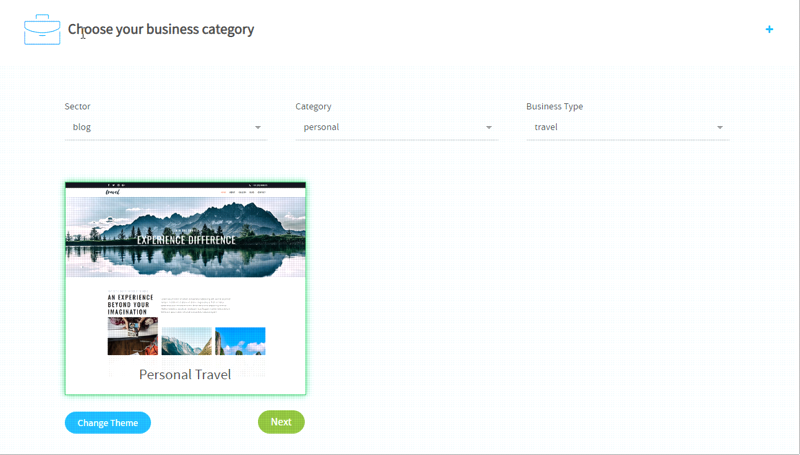This image is a screen capture showcasing a web interface with a predominantly white background and gray font. At the top of the image, there is a small blue briefcase icon next to the text "Choose your business category" in black. A gray mouse cursor is visible nearby, along with a blue plus sign.

Below this section, there are three gray submenus labeled as follows: 
1. **Sector:** Blog
2. **Category:** Personal
3. **Business type:** Travel

Further down, an image outlined in lime green features white text that reads "Experience Difference." The image depicts a scenic view with blue mountains, forest green trees, and a body of water reflecting light. It has a black border at the top and includes several submenus positioned above the image.

Continuing downward, the text "An experience beyond your imagination" is displayed alongside a slightly blurry picture, making the details difficult to discern. Adjacent to this picture, there is a paragraph or two of black text.

Additional nature photos are displayed underneath, including an image of mountains and another with blue skies, white clouds, and a partial view of what appears to be two people's heads. Below these images, the text "personal travel" is shown in gray.

At the bottom of the screen capture, two boxes are visible: a blue box with the text "Change theme" in white and a green box with the text "Next" in white.